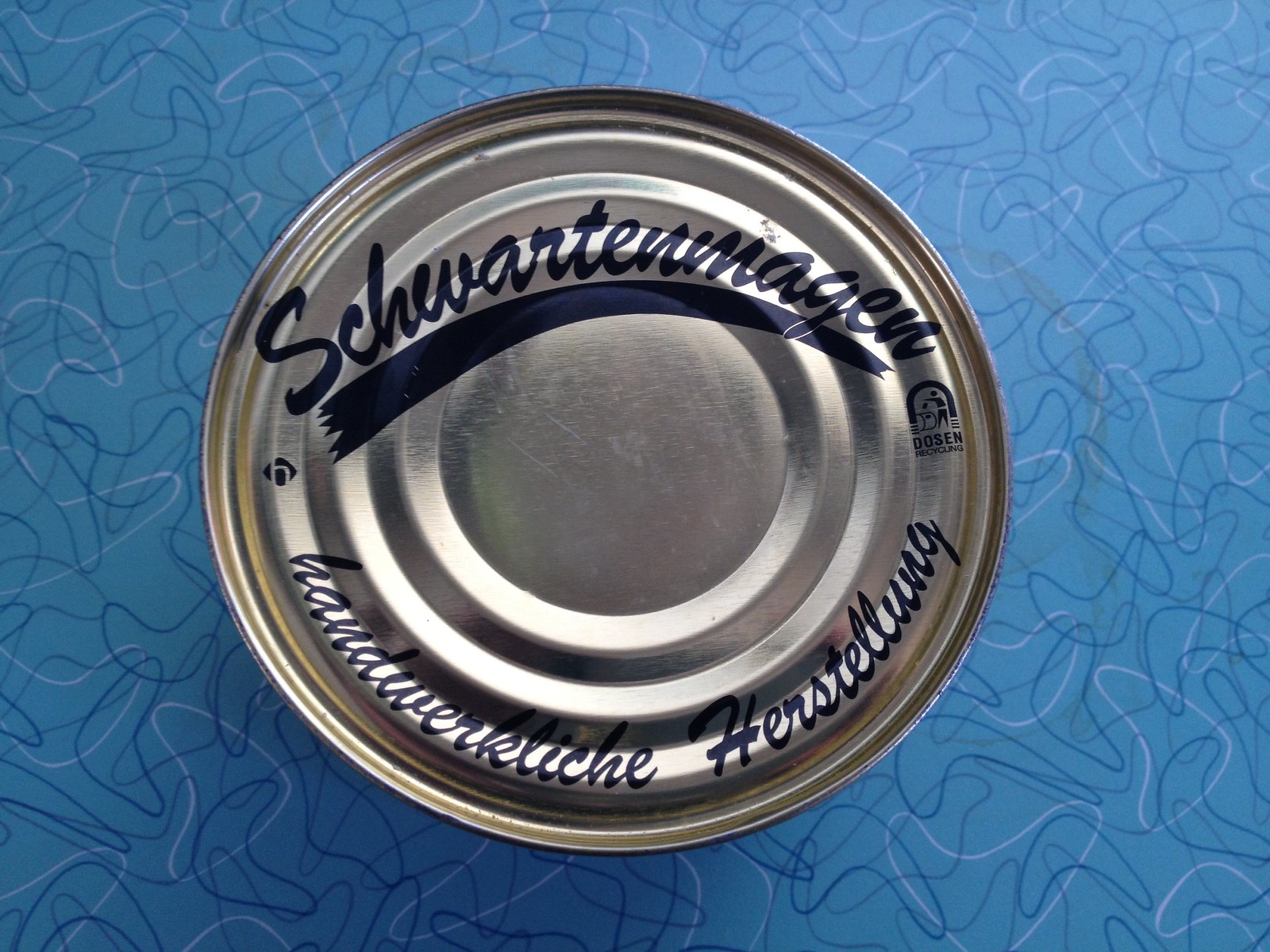In the foreground of the image, a tin can is displayed from a top-down perspective, revealing its circular shape and the embossed text on its lid. The text on the can reads "Schwartz and Megan," and below this, a phrase in German is printed: "Handwerkliche Herstellung." The background features a Formica tabletop in a sky blue color, adorned with a white, boomerang-like squiggly pattern that adds a whimsical touch to the scene. The overall composition blends the industrial feel of the tin can with the playful design of the retro-inspired countertop.